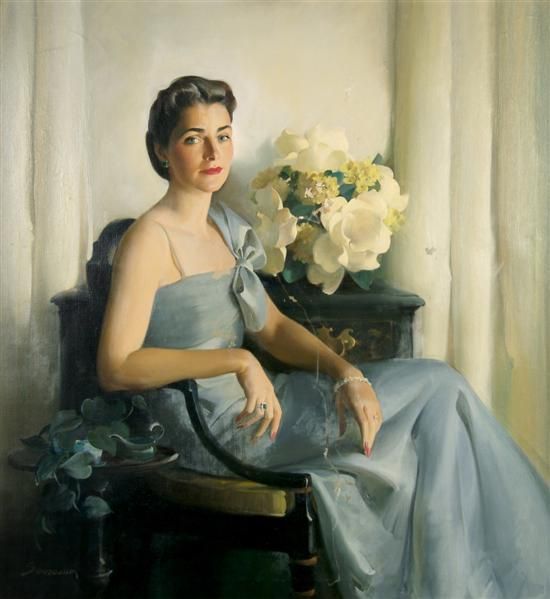This exquisitely detailed painting, rendered with such smoothness that no brushstrokes are visible, portrays a woman seated gracefully in an indoor parlor setting. The woman is adorned in a light, airy blue evening gown. The gown features a thin white strap over her right shoulder and a large, elegant bow over her left shoulder, made of satin or silk material, draping down to her knees. Her hands rest delicately on the arms of a black wooden chair with a yellow seat cushion. Her hair, dark and pulled back in an updo, complements the sophistication of her appearance, further highlighted by her red lipstick and eye makeup.

On her left wrist, she wears a pearl bracelet, and a ring adorns her right hand. To her left, a small table supports a cascade of blue flowers, while over her right shoulder, a large bouquet of white and yellow flowers stands on a dark blue wooden dresser. The serene background features soft beige curtains and a matching wall, enhancing the warmth and elegance of the room. The composition suggests a scene filled with subtle light, emphasizing the soft textures and the delicate interplay of colors. The painting captures a moment of poise and beauty, evoking a timeless grace.